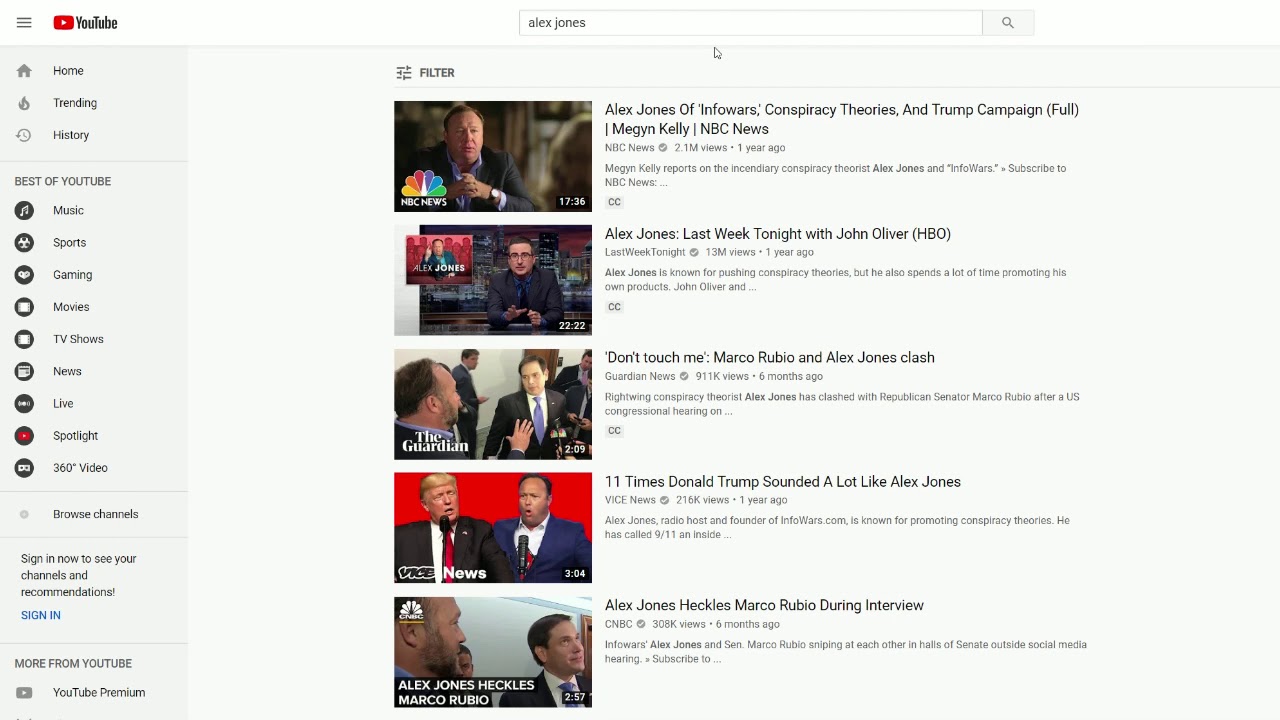Displayed in the image is a YouTube webpage featuring a prominent white border at the top with the YouTube logo in black. Below the logo, a white search bar with a gray outline appears, containing the search term "Alex Jones" written in black on the left side. Just beneath, in black text, are navigation options: "Home," "Trending," and "History," each separated by a gray line extending horizontally across the page.

Further down, the "Best of YouTube" section highlights various categories such as "Music," "Sports," "Gaming," "Movies," "TV Shows," "News," "Live," "Spotlight," and "360° Video," each followed by another thin gray line. Additional navigation options include "Browse Channels" and a prompt that reads, "Sign in to see your channels and recommendations!" The "Sign in" button is blue, accompanied by another thin gray line.

Below this, in gray text, there is a section titled "More from YouTube," which includes "YouTube Premium" written in black. On the right side of the page, a "Filter" option is available, also in black, placed above another thin gray line. A white mouse pointer is visible, placed underneath the middle part of the search bar.

The main content displays a list of video titles related to Alex Jones. The first video is titled "Alex Jones of the Info Wars, Conspiracy Theories and Trump Campaign Full" by Megan Kelly, NBC News, posted one year ago with 2.1 million views. The second video, from "Last Week Tonight with John Oliver," features Alex Jones, accumulated 13 million views after being posted one year ago. The third video titled "Don't Touch Me, Marco Rubio, Alex Jones Clash" by Guardian News has 911,000 views, posted six months ago. The fourth video is "11 Times Donald Trump Sounded a Lot Like Alex Jones." The final video title reads "Alex Jones Heckles Marco Rubio During Interviews."